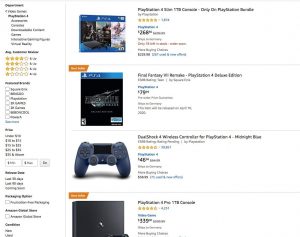The image displays a promotional page featuring various PlayStation 4 gaming bundles and accessories. Central to the layout is the PlayStation 4 Pro 1TB console, adorned in sleek black. Adjacent to it is the PlayStation 4 Slim 1TB console, also showcasing a sophisticated black finish. Highlighted prominently is a PlayStation 4 wireless controller, designed specifically for the PlayStation 4, in a bold blue color. The page also features the cover art of a PlayStation 4 disc for the game "Final Fantasy," marked by its distinctive artwork and branding. Surrounding these items are various ratings and textual information, though the specifics aren't clearly visible. The color scheme of the page includes black, blue, gray, and orange accents that emphasize the gaming products and their appeal.